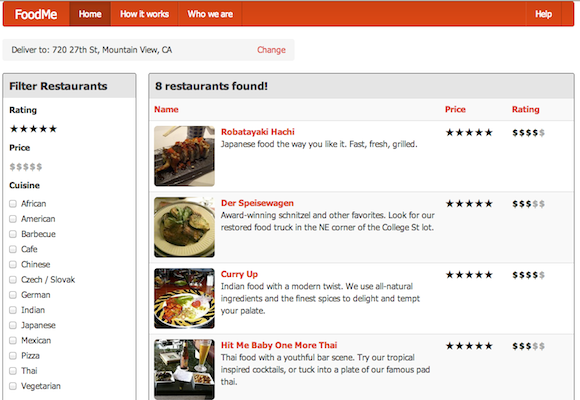The website page features a rich layout against an orange rectangular background with various menu options and information in white text, except for a "Home" button displayed on a burgundy rectangle. The menu options include "Food," "Me," "Home," "How It Works," "Who We Are," and "Help." There's an address field displaying the delivery location as "720 27th Street ST, Mountain View, CA," accompanied by an orange "Change" button.

The interface allows users to filter restaurants by rating, price, and cuisine type. The rating filter displays five stars, while the price filter shows five dollar signs. Cuisine options, each with an adjacent checkbox, include African-American, Barbecue, Cafe, Chinese, Chef Slovak, German, Indian, Japanese, Mexican, Pizza, Thai, and Vegetarian.

The search results reveal eight restaurants. Each entry includes the restaurant's name, price range, rating, and an accompanying image. For instance, "Repati Hachi ROBATAYAKI" displays a five-star rating and a price tag of four out of five dollar signs, along with its image. Another restaurant, "Dear Speisewagen," shows a five-star rating and a price tag of three dollar signs, with its image positioned beneath the name.